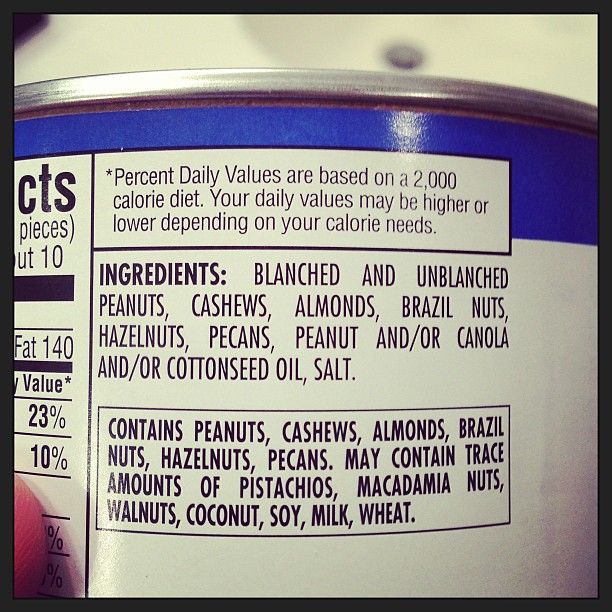The image depicts a detailed close-up of a food can label, primarily focusing on the ingredients list and partial nutrition facts. The ingredients, prominently centered, list blanched and unblanched peanuts, cashews, almonds, Brazil nuts, hazelnuts, pecans, peanut and/or canola and/or cottonseed oil, and salt. Below this list, there's a warning label indicating that the product contains peanuts, cashews, almonds, Brazil nuts, hazelnuts, and pecans, and may contain trace amounts of pistachios, macadamia nuts, walnuts, coconuts, soy, milk, and wheat. The upper section of the label features a blue band while the rest of the label has a white background. On the far left, the edge of the nutrition facts section is visible, showing fat calories as 140 with more details obscured. A small part of a person's thumb is visible in the lower left corner, which appears to be of a Caucasian person. Above the ingredients, a disclaimer notes that the percent daily values are based on a 2000 calorie diet.